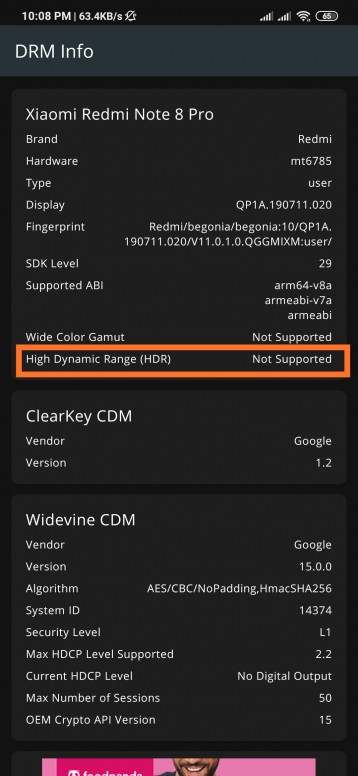**Detailed Description of the Mobile Device Information Screen:**

The image displays a mobile device's settings screen, detailing specific system information. The backdrop of the screen is a dark gray color, with a lighter gray header bar. The header bar, in medium gray, prominently displays "DRM INFO" in all capital letters.

At the top of the screen, basic device information is visible. The time is shown as 10:08 PM, and a data speed indicator reads 63.4 kbps. The notification bell icon indicates notifications have been turned off. To the right, two signal graphs are present, each showing four to five bars, suggesting strong connectivity. A full Wi-Fi signal icon and battery status at 65% are also displayed.

Beneath the header, further details about the device are listed:
- **Device:** Xiaomi Redmi Note 8 Pro
- **Brand:** Redmi
- **Hardware:** MT6785
- **Type:** QPIA.190711.020
- **Fingerprint:** [There is additional, extensive data on the fingerprint that is not fully spelled out here]

The section continues with:
- **SDK Level:** 29
- **Supported ABI:** 
    1. arm64-v8a 
    2. armeabi-v7a 
    3. armeabi

The screen also includes a summary of multimedia capabilities:
- **Wide Color Gamut:** Not Supported
- **High Dynamic Range (HDR):** Not Supported

These unsupported features are highlighted by an orange rectangle around the text.

Below this, there is a lighter blue section detailing DRM-related information:
- **Clear Key CDM:** 
    - **Vendor:** Google 
    - **Version:** 1.2
    
Following this, information regarding Widevine CDM is provided, including various options such as:
- **Vendor:** 
- **Version:**
- **Algorithm:**
- **System ID:**
- **Security Level:**

Each of these attributes has corresponding details listed to the right, filling out the specific capabilities and parameters of the device's DRM support.

The careful arrangement of colors and highlights enhances the clarity of distinguishing between supported and unsupported features.